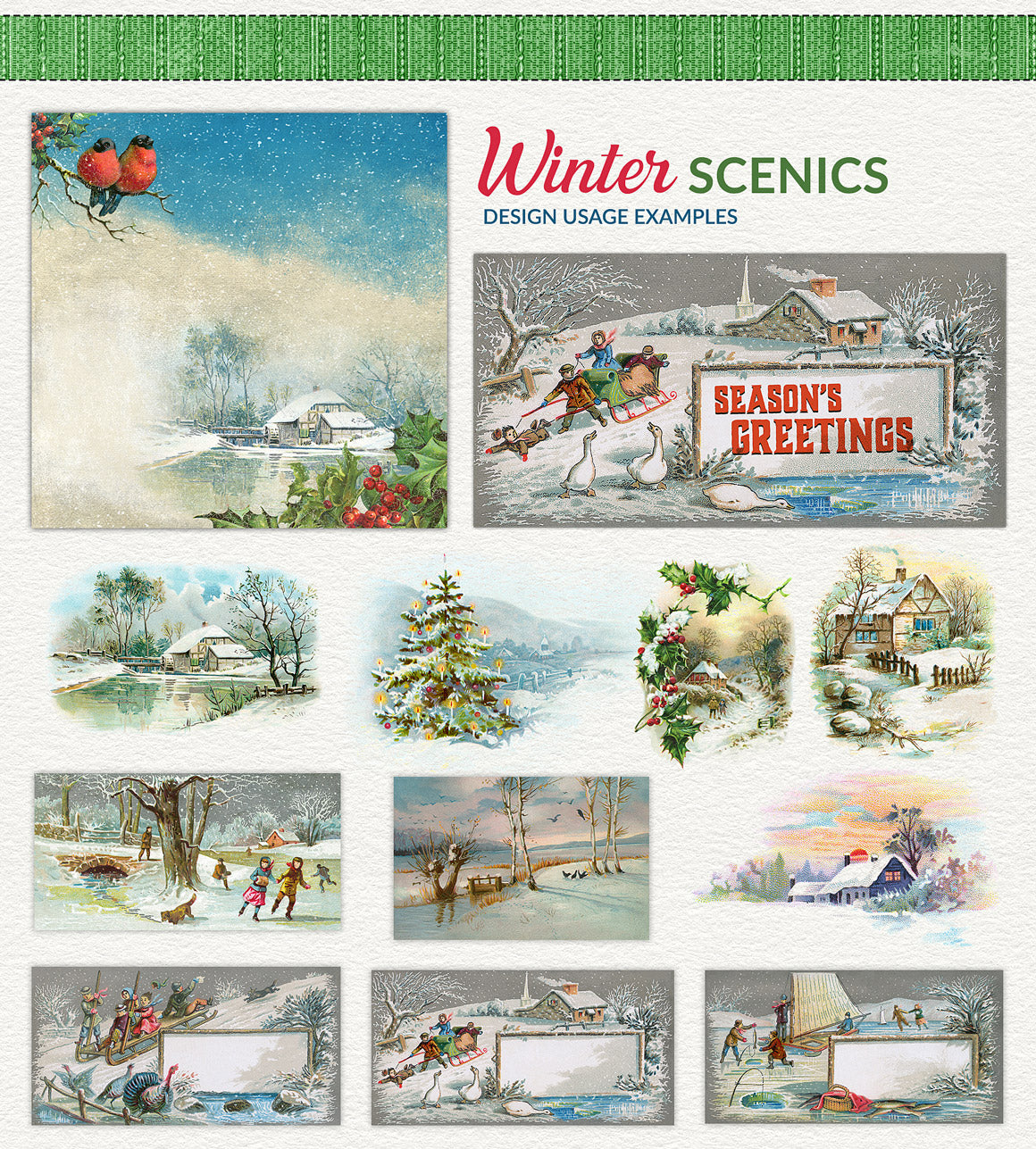The image depicts a display that appears to be either the back of stationery or a packaging for Christmas cards, titled "Winter Scenics Design Usage Examples." The display showcases twelve different photos arranged in a grid, with two large photos on the top row, followed by four smaller photos, then another four, and finally two rows of three photos each. Each photo highlights a winter or festive scene, including kids sledding and skating on a frozen pond, Christmas trees, homes by lakes, children boating, and a picturesque house on a frozen lake adorned with red birds and holly with red berries. Other elements include a turkey in one photo and a dog in another. To the right of the images, there's text saying "Seasons Greetings," emphasizing the holiday theme of the collection.